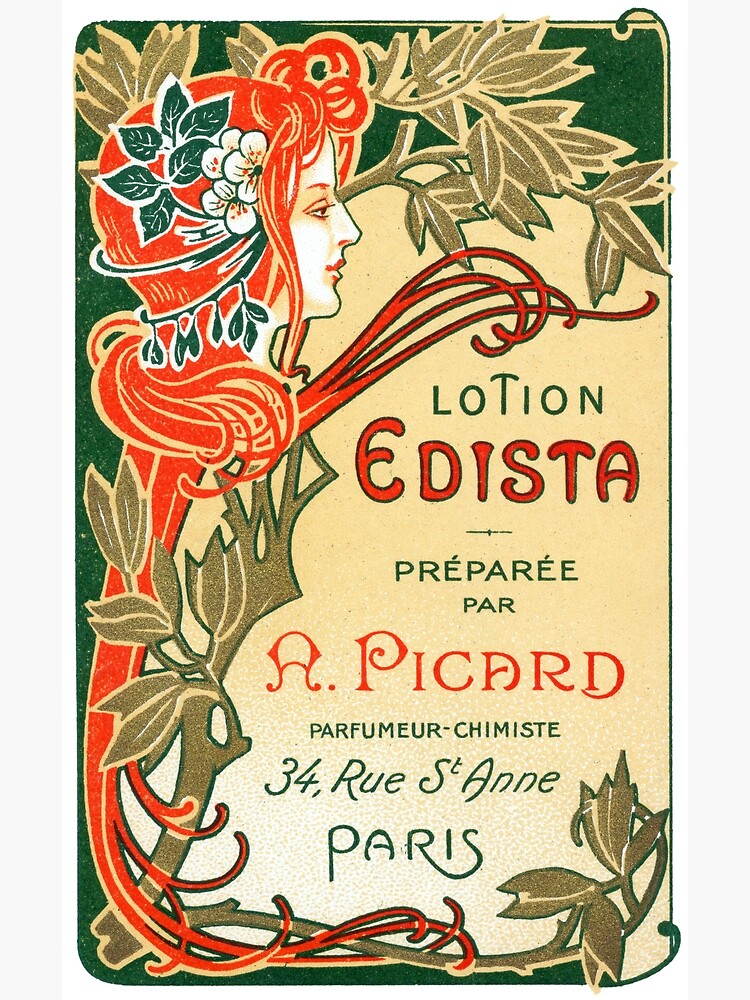The image in question is a vintage-style advertisement poster for lotion, featuring a predominantly tan background accented with black or dark green edges, especially along the top and left side. Taking center stage is an artistic drawing of a woman's profile, showcasing her strikingly bright red hair adorned with an array of flowers and leaves. Her vibrant hair cascades down alongside the left side of the image, intertwined with tentacle-like red extensions and pale green leaves. The poster bears the inscription "Lotion Edista" prominently to the right of the woman's image, followed by the text "Preparé Par A. Picard, Perfumer Chimiste, 34 Rue Saint Anne, Paris," each line presented in distinctive fonts and colors — green and red. The combination of beige, pale green, pale red, black, and white hues throughout the design reinforces its vintage aesthetic.